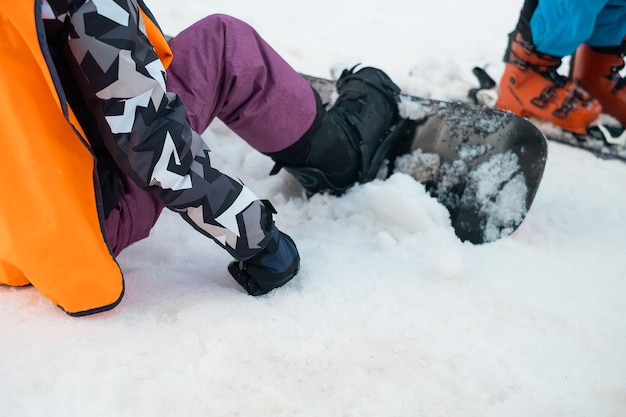This detailed photograph captures the scene of a snowy slope featuring a snowboarder in the foreground, seated on the ground. The snowboarder is clad in a bright orange overvest layered over a black, gray, and white geometric patterned shirt. Their hands are protected by blue gloves, and they are wearing vibrant purple snow pants paired with black snow boots. Their black snowboard, attached to their boots, is propped up with a small mound of collected snow behind it near their foot.

In the background, the lower half of another individual is visible, presumably a skier. This second figure is dressed in blue pants and distinct bright orange ski boots, with only their legs, feet, and a part of their skis captured in the frame. The snowy terrain envelops both individuals, emphasizing the winter sports setting. The photo notably omits their faces, focusing instead on their gear and positioning on the snow.